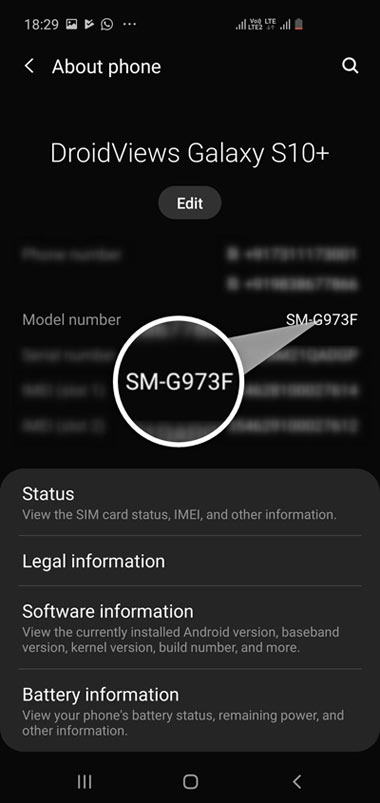The image depicts a smartphone screen displaying an "About Phone" menu for a Samsung Galaxy S10+. At the top of the screen, there are a Wi-Fi icon and a battery icon. Below these icons, there is a left-facing arrow labeled "About Phone," and to the right of this label, there is a search icon. 

Further down, the text "Droid Views" followed by "Galaxy S10+" is displayed in a single line. Directly beneath this, there is an edit button. Under the edit button, a circular icon encloses the text "SM-G973F," which is identified as the model number of the device. 

The screen is divided into several sections: 
1. **Status:** Provides the status of the SIM card, IMEI, and other relevant information.
2. **Legal Information:** Stores the legal documentation and disclaimers.
3. **Software Information:** Offers details about the currently installed Android version, band-based version, kernel version, build number, and more.
4. **Battery Information:** Displays the phone's battery status, remaining power, and additional battery details.

At the very bottom of the screen, there is a banner with a drop-down icon, a home button, and a left-facing arrow.

This level of detail ensures a comprehensive understanding of the screen layout and the functionalities available in the "About Phone" menu of the Galaxy S10+.